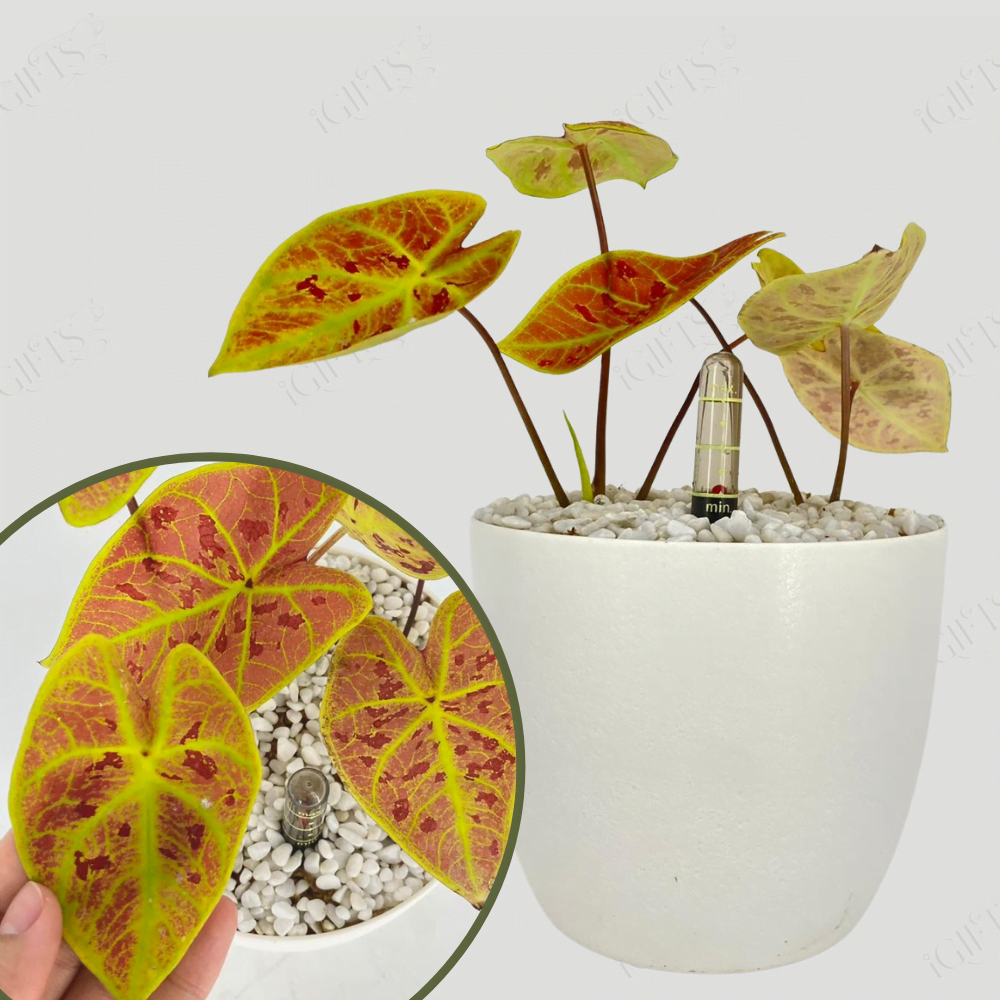The image is a detailed color photograph in portrait orientation, capturing a white, ceramic-looking plant pot with white gravel inside. The pot is slightly to the right of center and widens at the top. Emerging from the pot are about five stems with large, pointed oval leaves. The leaves vary in color, displaying shades of green and orange with distinct green veins. Notably, two of the leaves are primarily green, while two others are mainly orange with green veins, and some leaves exhibit darker red blotches. In the middle of the pot, there is a clear glass moisture indicator with yellow measurement bands and a black stripe labeled "MIN" in gold at the bottom. The photograph also features an inset section at the lower left, providing a top-down view of another pot, where three orange leaves with green veins are visible. A hand is seen holding one of these leaves, offering a closer look at the detail and colors. The style of the photograph aligns with representational realism, focusing on the precise and true-to-life depiction of the plant and its elements.